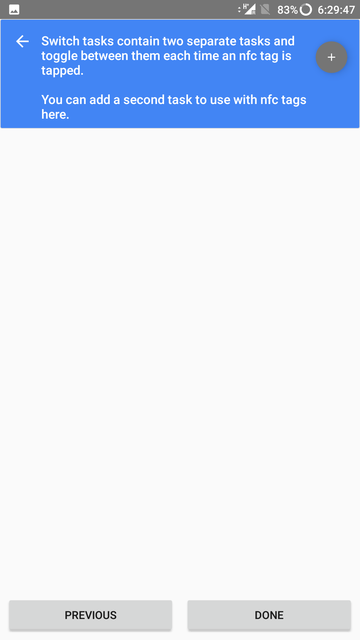At the top of the medium gray bar, there is a white square on the left with two small gray dots inside it. To the right, the battery level is displayed as 83%, alongside a white circle that nearly forms a complete loop, missing about half an inch near the upper left part. Next to the battery icon, the time is displayed as 6:29:47. A small white arrow pointing left is inside a blue square to the right of the time, followed by the text: "Switch tasks between two separate tasks each time an NFC tag is tapped." An inch below that, the text reads: "You can add a second task to use with the NFC tags here," with a gray circle containing a white plus sign to the right of this text. About six inches below, there are two small gray rectangles. The first rectangle contains the word "PREVIOUS" in black capital letters, while the second rectangle holds the word "DONE," also in black capital letters.